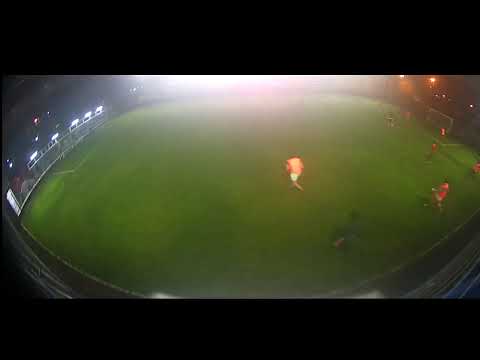This photograph showcases a blurry, fisheye view of a soccer match captured from an elevated perspective. The green grass field is framed by horizontal black strips at the top and bottom, and is illuminated by an array of bright white lights, five of which are clearly visible on the left side of the image. The brighter light source from the top further intensifies the scene. Players can be seen in orange shirts and white shorts, with six visible players concentrated mostly around the right goal, two of whom are positioned directly in front of it. One player stands notable near the center of the field. The field appears devoid of any markings or lines, intensifying the focus on the players and the game in progress. The image captures the essence and dynamic atmosphere of the match despite the low image quality.